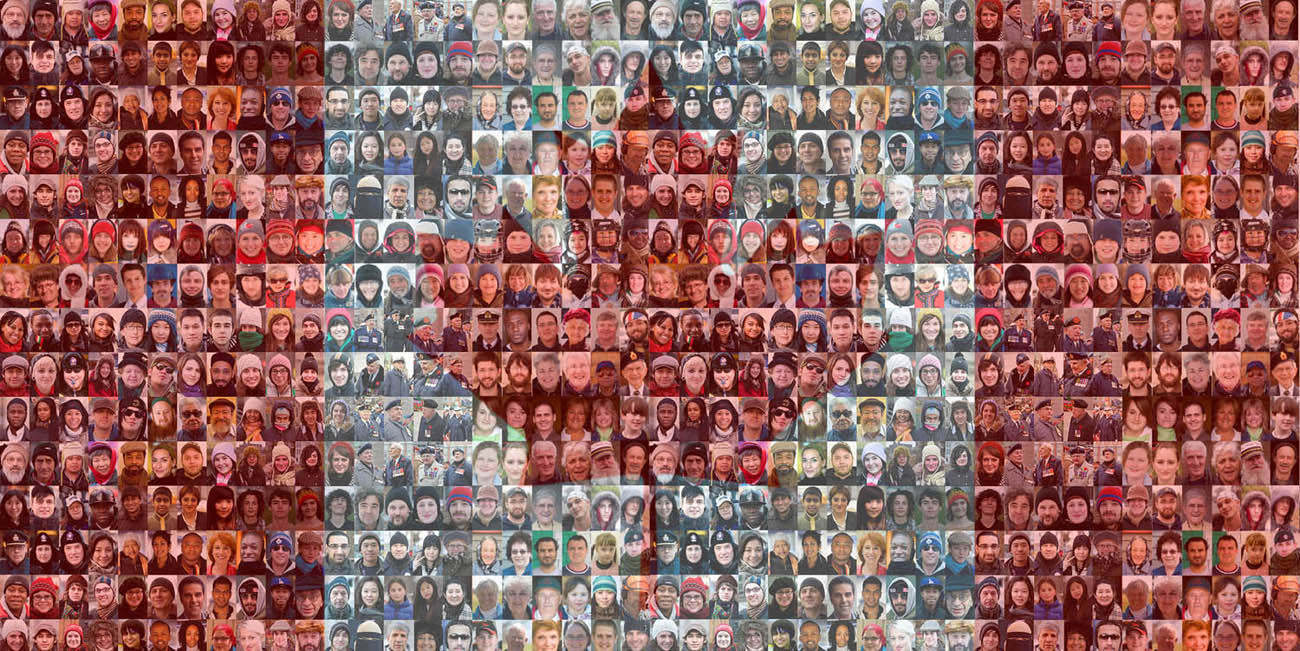The image is a unique and meticulously crafted mosaic of the Canadian flag, composed entirely of individual portrait photos, displaying a diverse array of faces. The flag, rectangular and horizontally oriented, showcases the iconic design with two vertical red bars on the left and right sides and a central white square. In the center of this white section lies a red maple leaf, also created from a collection of these tiny headshots. Each face represents a person from various walks of life, encompassing different ages, genders, and ethnic backgrounds, symbolizing the rich diversity of Canada. The photos are carefully tinted to match the flag's colors: the portraits on the red sections have a red hue, those in the white area are lighter, and the faces forming the maple leaf are also tinged with red. Notable details include a man with a white beard and a beanie located in the top left corner and another man smiling while wearing a beanie in the bottom right corner. The sheer number of faces, likely numbering in the hundreds or even thousands, creates an intricate and vibrant representation of the Canadian flag, celebrating the multitude of individuals that make up the fabric of the nation.